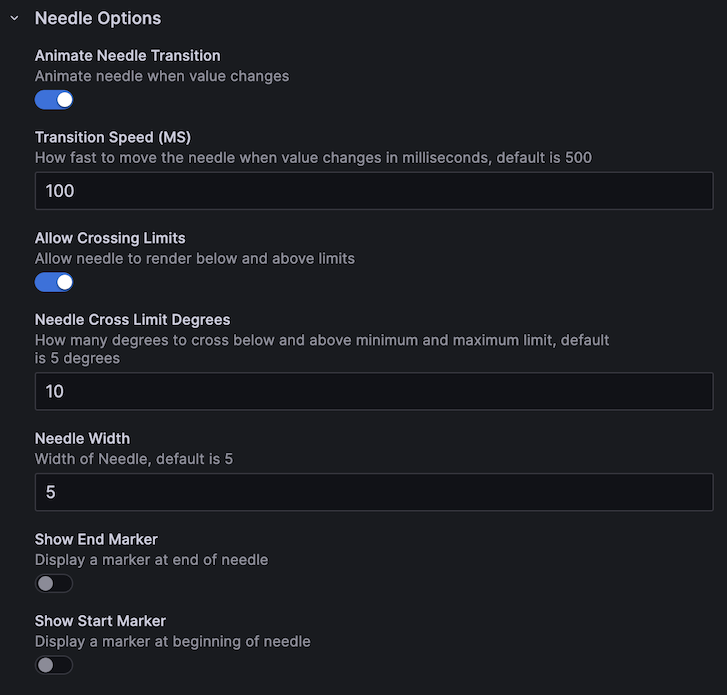The image showcases a section of a website with a black background, prominently featuring "Needle Options" in white at the top. 

Under "Needle Options," the following settings are displayed:

1. **Animate Needle Transition**: This toggle, accompanied by a blue slider with a white circle, is activated. Below, it specifies "Animate needle when value changes."
   
2. **Transition Speed**: Detailed description of how fast the needle moves when the value changes, measured in milliseconds. The default value is 500ms, but the current setting is 100ms.

3. **Allow Crossing Limits**: This setting is also toggled on, using a blue slider with a white circle. It explains that this option permits the needle to render below and above the specified limits.

4. **Needle Cross Limit Degrees**: This setting defines how many degrees the needle can cross below or above the minimum and maximum limits. The default is five degrees, but the current configuration is set to ten degrees.

5. **Needle Width**: Specifies the width of the needle with a default value of five, which is also the current setting.

6. **Show End Marker**: Describes the option to display a marker at the end of the needle. This is currently turned off.

7. **Show Start Marker**: Describes the option to display a marker at the beginning of the needle. This is also turned off.

There are no additional images or context provided to clarify what specific application or purpose these needle settings pertain to.